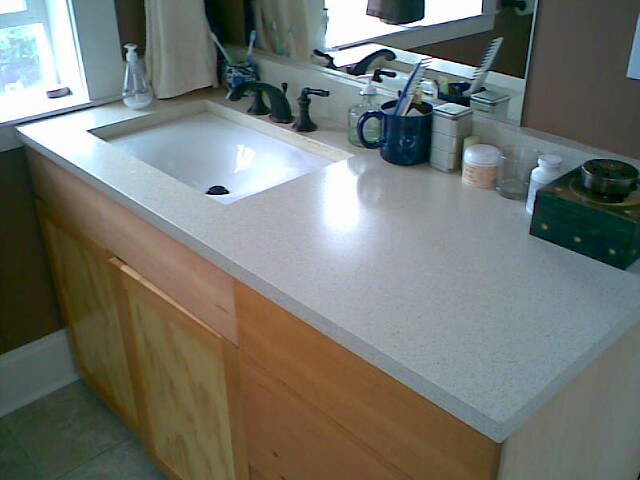The photograph captures an old bathroom counter space, evident from its grainy texture and dated coloring. The counter is a broad, rectangular surface with a white sink positioned towards the left. The sink has a black spout accompanied by two individual handles, one on each side. To the left of the sink, a soap bottle and a cup containing two toothbrushes are neatly placed. On the right side of the sink, a mug holding a comb and other indistinct items is visible. Further right, there are multiple containers, likely filled with cotton swabs, and a small jar that appears to contain lotion. At the extreme right end of the counter, a green box possibly intended for jewelry storage sits, topped by a bowl that may also serve a similar purpose. Below the counter, brown wooden cabinet doors suggest additional storage space.